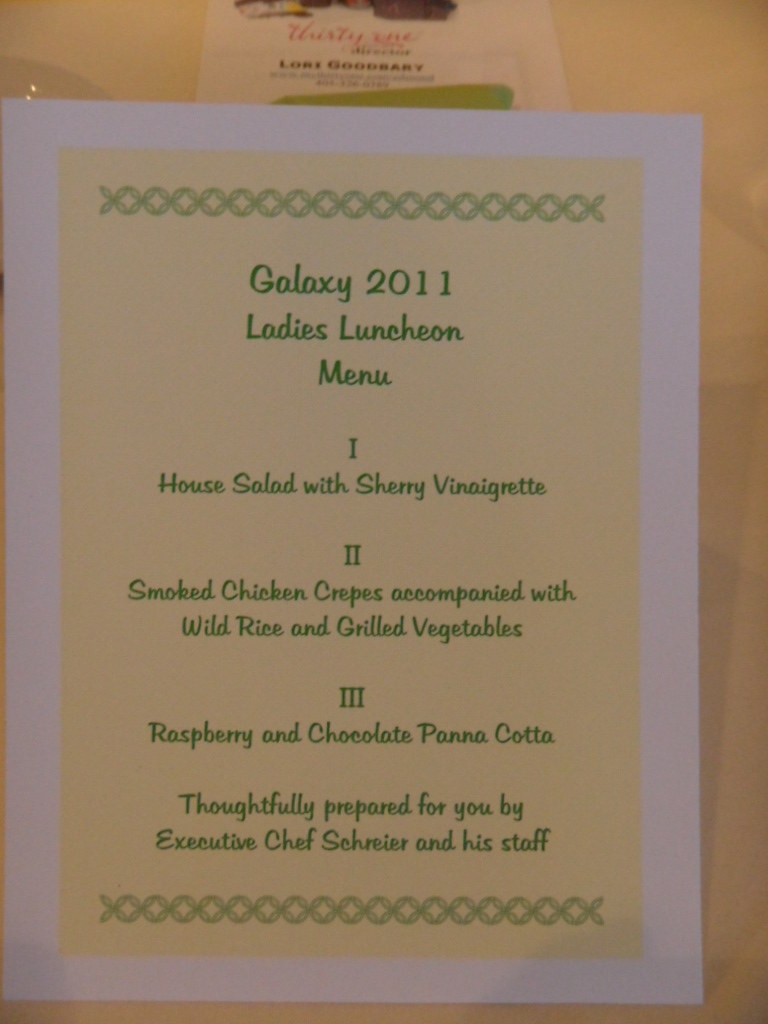The image depicts a lunch menu from the Galaxy 2011 Ladies Luncheon, elegantly presented on a white piece of paper placed against a brown background, possibly a table. The menu itself is formatted as a vertical rectangular-shaped yellow-beige label with green text. At the top, there is a decorative horizontal line consisting of small green O's flanked by X's on either end. Below this decorative line, in cursive script, it says "Galaxy 2011 Ladies Luncheon Menu."

The menu features three items, each listed with Roman numerals:
  I. House salad with sherry vinaigrette
  II. Smoked chicken crêpes accompanied by wild rice and grilled vegetables
  III. Raspberry and chocolate panna cotta

Following the list of dishes, a note reads: "Thoughtfully prepared for you by Executive Chef Schreier and his staff." This message is also in green text. At the bottom, a similar decorative line mirrors the one at the top, featuring small green O's with X's at the ends. There is an additional piece of text outside the menu borders at the top, but it is too small to be deciphered.